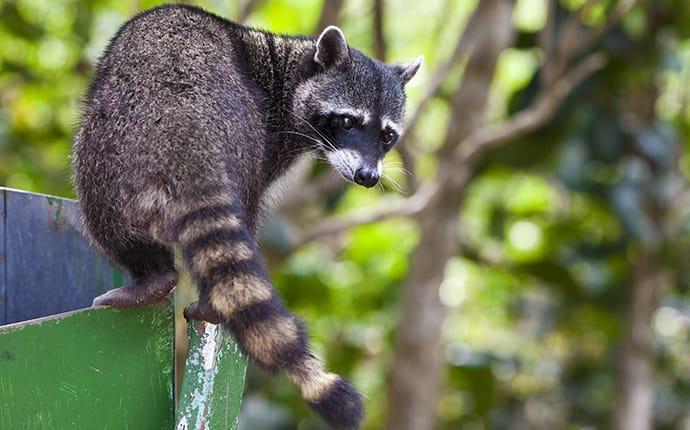In a horizontal, rectangular photograph, a raccoon is perched on the left side atop a green-painted, round metal object that resembles either a trash can or a barrel. The object reveals a silver-gray interior. The raccoon is standing with its back to the camera, but its head is turned to face the viewer. It features distinctive black and gray fur, with a black "mask" around its eyes, a black nose, ears sticking up, white whiskers, a white snout, and a hint of white above its eyes. The raccoon's tail displays alternating brown and black rings, and its back feet are clearly visible. The background is blurred, featuring green leaves bathed in sunlight and tree branches crossing the frame, enhancing the natural setting of this sunny day.